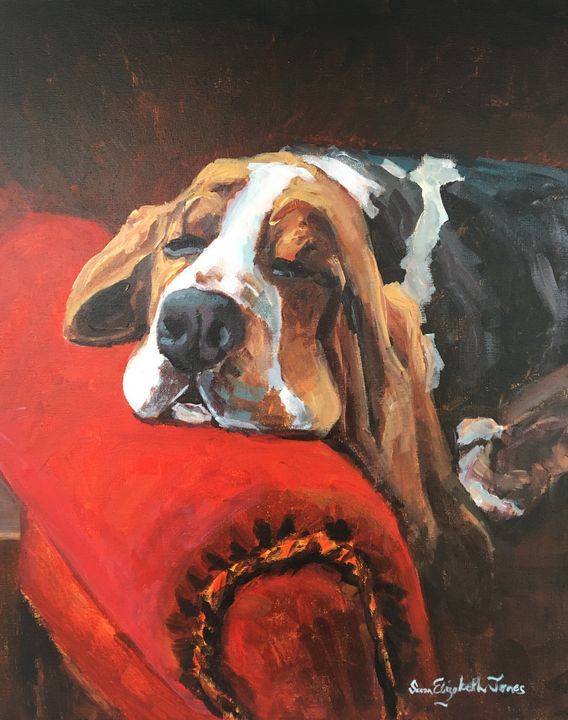This detailed painting captures a hound dog, characterized by its long, floppy brown ears and distinct coloration. The dog, with its head resting on the large arm of a deep red cloth sofa, appears to be taking a nap with its eyes closed and mouth slightly drooping. Its fur is a blend of brown, white, and black, with a memorable white stripe running down its nose and around its snout. The dog's body transitions to black towards its rear. The background is an abstract mix of brown splotches, adding depth to the portrait without detracting from the central figure. The artist has signed their name, "Susan Elizabeth Jones," in white paint at the bottom right corner of the painting. Overall, this painting evokes a sense of calm and restfulness, spotlighting the sleeping dog on a richly colored sofa.